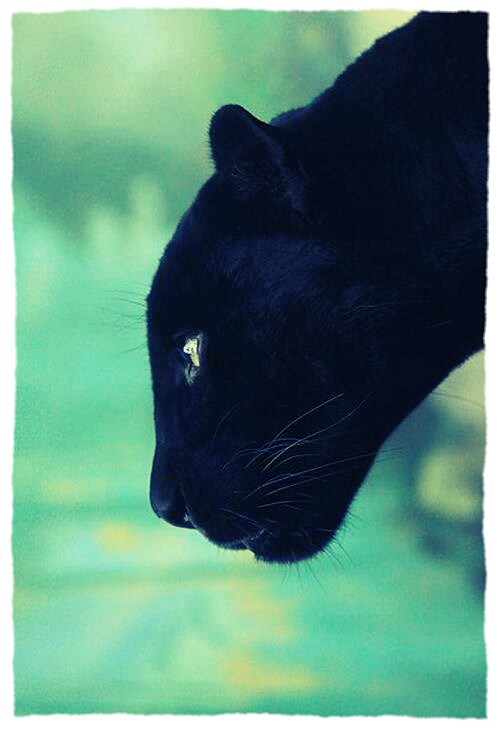The photograph captures a stunning side profile of a black panther's head, with the focus exclusively on the panther. The panther's sleek black fur looks soft and glossy, contrasting beautifully with its piercing yellow eyes that are directed to the left. This arresting image shows only from the neck forward, highlighting the left side of the head and neck. The panther's snout is adorned with multiple white whiskers, while additional black whiskers sprout above its eyes, adding to its majestic appearance. The overall composition is heightened by the blurred background, which is an indistinct blend of green and blue hues, possibly suggesting a forest or jungle, yet remaining ambiguous and abstract. The panther's head is slightly tilted downwards, which might imply it is lowering its head to drink water. The panther's ears are positioned above the nose, adding depth to the diagonal orientation of its profile, capturing a moment that feels very real and lifelike despite the artistic quality of the image.